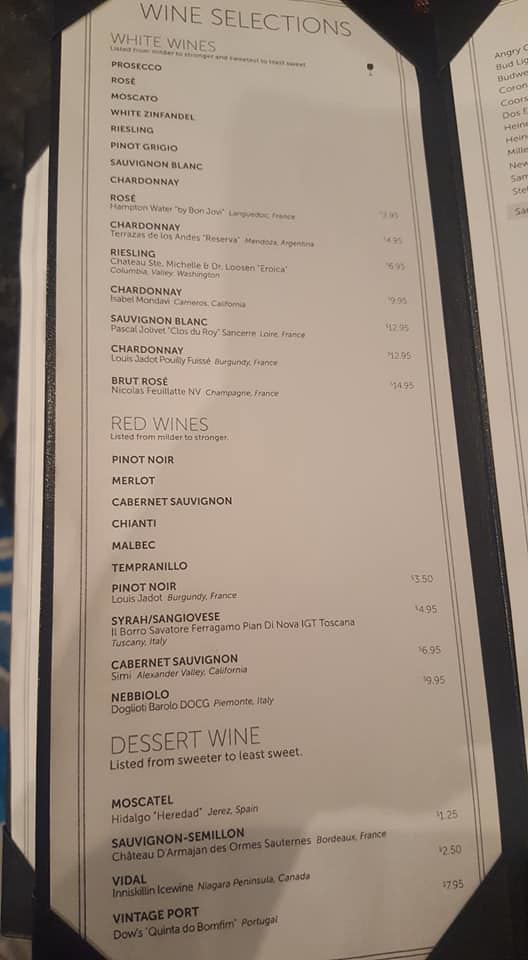The photograph features a detailed wine menu encased in a sleek black binder. The menu is presented on a long piece of white paper, securely tucked into the corners of the binder, adding to its neat and formal appearance. A shadow partially obscures the page, giving it a slightly mysterious, yet elegant ambiance.

At the top of the menu, the heading "Wine Selections" is prominently displayed. Below this, the list begins with the category "White Wines," showcasing a variety of selections: Prosecco, Rosé, Moscato, White Zinfandel, Riesling, Pinot Grigio, Sauvignon Blanc, and multiple entries of Chardonnay, interspersed with other wines like Brut Rosé. 

To the right of each wine name, the prices are neatly aligned, providing a clear and concise overview for patrons. Following the white wines, the next category listed is "Red Wines," featuring a robust selection including Pinot Noir, Merlot, Cabernet Sauvignon, Chianti, Malbec, Tempranillo, Syrah, Sangiovese, and Nebbiolo, each with corresponding prices to the right.

At the bottom, the "Dessert Wine" category is delineated, organized from sweeter to least sweet. This section includes Moscatel, Sauternes, Vidal, and Vintage Port, giving a comprehensive look at the wine offerings for those with a penchant for sweeter finishes.

To the right of the current page, a sliver of the next page is visible, hinting at the continuation of the extensive wine list. The meticulous organization and variety suggest a well-curated selection, aimed at catering to diverse palates and preferences.